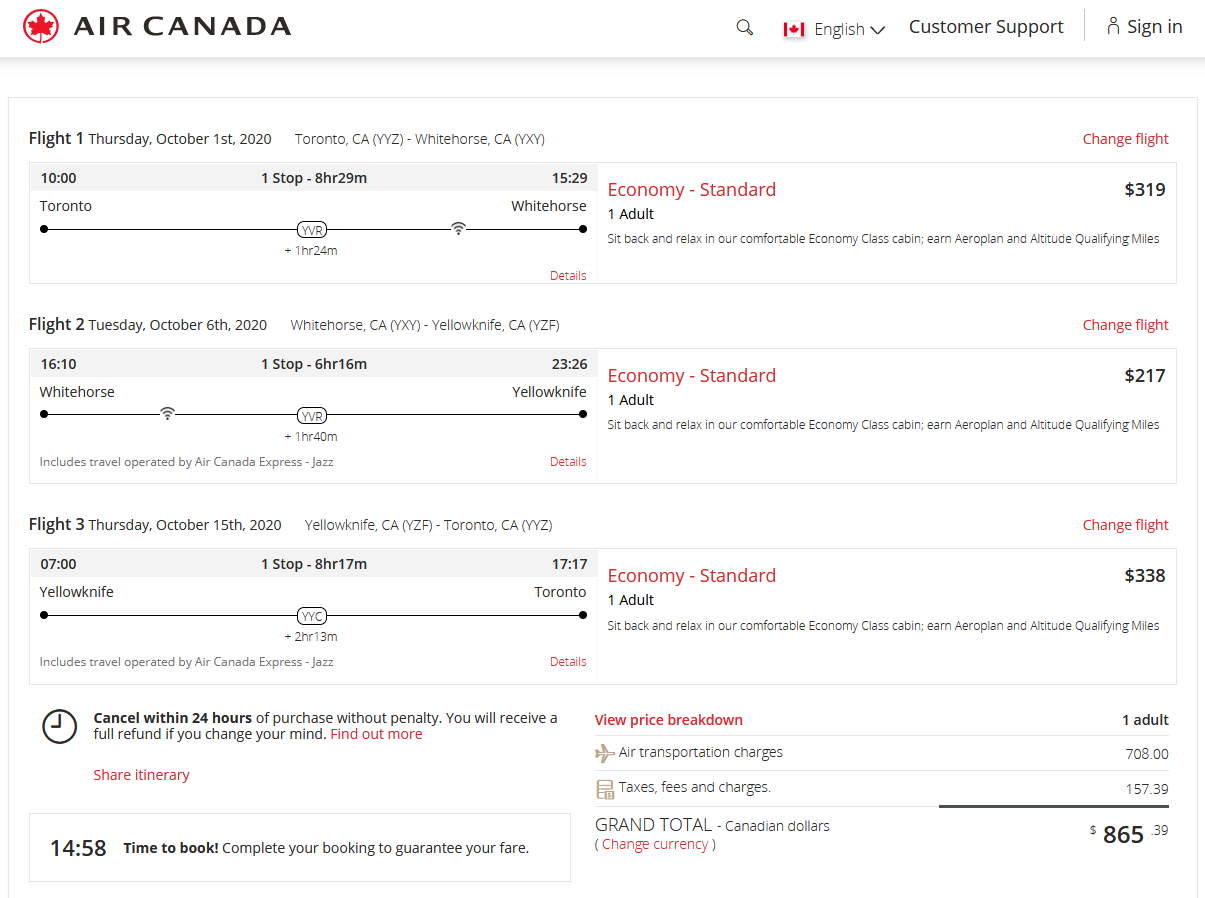This detailed caption describes a flight schedule from Air Canada:

"In this screenshot of an Air Canada flight itinerary, the Air Canada logo, a distinctive red maple leaf encircled by a red outline, is prominently displayed in the upper left corner. Next to the logo, 'Air Canada' is clearly written. The user interface also features a search option, a language setting currently set to English, customer support, and a sign-in option.

The schedule outlines three flights. The first flight is on Thursday, October 1, 2020, from Toronto Pearson International Airport (YYZ) to Erik Nielsen Whitehorse International Airport (YXY). The departure time from Toronto is 10:00 AM, with one stop along the route. The total travel time is 8 hours and 29 minutes. This economy standard flight is priced at $319 for one adult, and includes the comfort of Air Canada's economy class cabin, where passengers can earn Aeroplan and Altitude Qualifying Miles.

The second flight is scheduled for Tuesday, October 6, 2020, departing from Erik Nielsen Whitehorse International Airport (YXY) to Yellowknife Airport (YZF). This flight, also in economy standard for one adult, is priced at $217. Passengers will enjoy the comfortable economy class cabin and the opportunity to accrue Aeroplan and Altitude Qualifying Miles.

The final flight listed is on Thursday, October 15, 2020, from Yellowknife Airport (YZF) to Toronto Pearson International Airport (YYZ). The fare for this economy standard flight for one adult is $338. Similar to the other flights, this service offers a relaxing experience in Air Canada's economy class cabin with the added benefit of earning Aeroplan and Altitude Qualifying Miles."